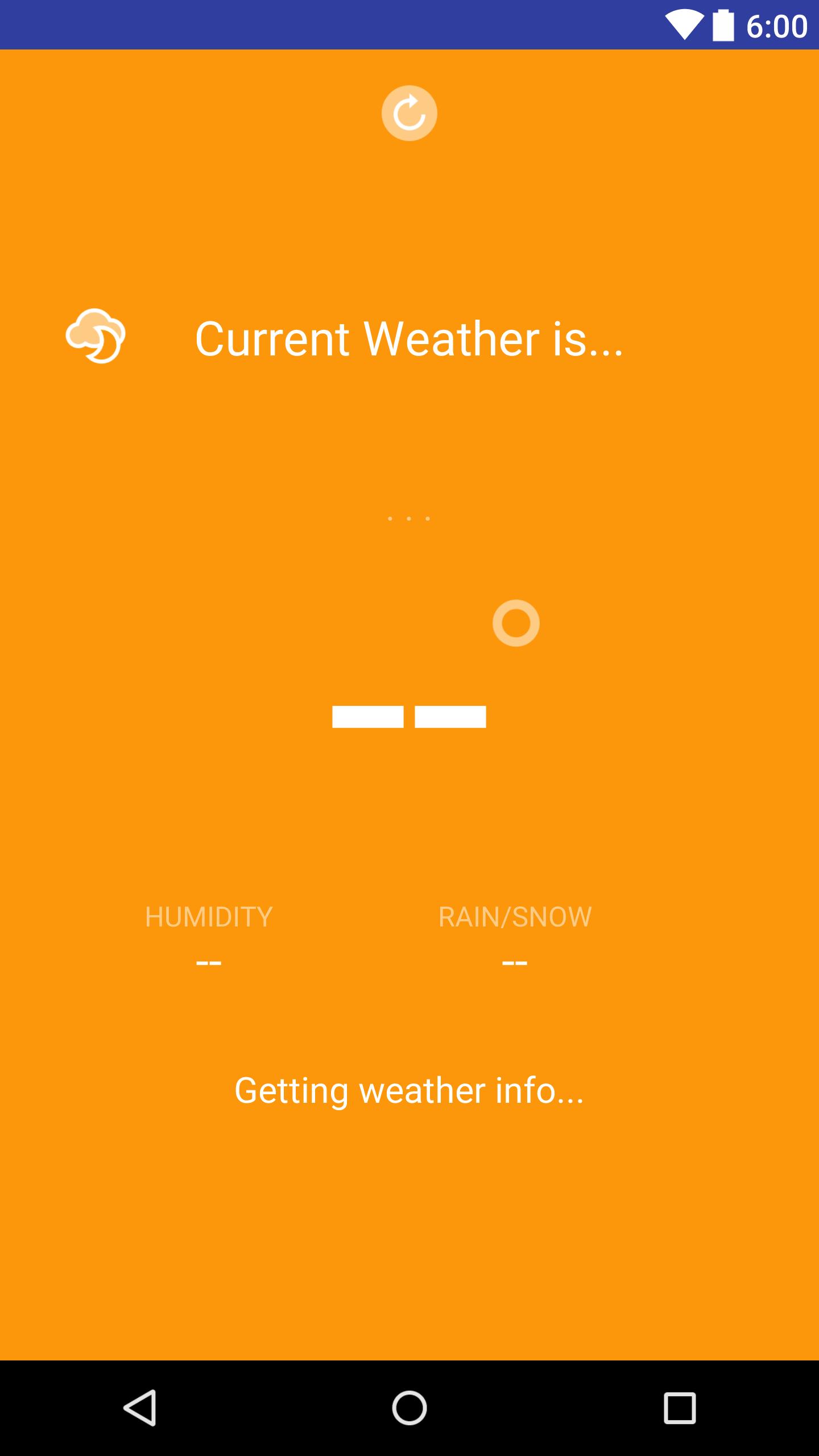This image is a screenshot taken from a cell phone, illustrating a weather application interface. At the very top of the screen, a blue status bar spans horizontally, displaying white icons for signal strength and battery life in the top right corner. The time is indicated as 6:00.

The main portion of the screen features an orange background. Near the top, a refresh button is visible, depicted as a circular arrow icon. Below this, there is a white text line stating "Current weather is...". To its left, an icon of a cloud with a superimposed moon provides a suggestive representation of a nighttime weather condition.

Beneath this icon, a small hollow circle is present, followed by two bright white dash-like rectangles, which stand out more prominently than other elements on the screen. Further below, the text "Humidity" is displayed, with two dashes underneath it. To the right of this section, another label reads "Rain/Snow" with two dashes beneath it as well. The phrase "Getting weather info..." appears in white letters, hinting at ongoing data retrieval.

The bottom of the screen features a black navigation bar with three icons: a back arrow, a circle, and a square, providing standard navigation options typical to many mobile interfaces.